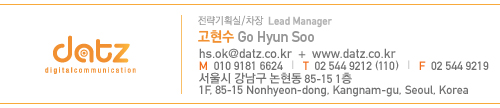The image depicts a section that resembles the bottom of an email signature, framed with thin orange lines at the top and bottom and featuring a vertical thin orange line separating two sections. On the left side, in bold, funky orange letters, it reads "D-A-T-Z," with "Digital Communication" in smaller orange print beneath it, creating a distinct logo-like appearance. On the right side, there is a detailed black and light gray text layout that includes orange highlights. The first line reads "Lead Manager" followed by Korean characters, and beneath it, the name "Go Hyun Soo" is displayed. Below this, there is a series of contact details including an email address, website, telephone number, fax number, mobile number, and a street address, all situated in Seoul, Korea. The text primarily uses black print, with certain elements like characters and numbers in orange, all set against a white background.